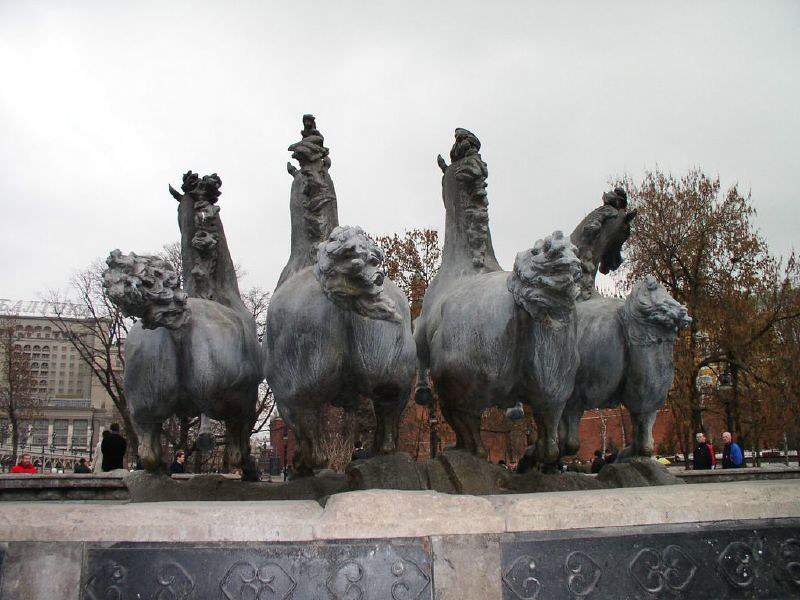This outdoor photograph captures a detailed view of a remarkable statue composed of four horses, positioned at the center of a circular area resembling that of a college campus. The horses, rendered in a typical metallic gray often seen in outdoor sculptures, are mounted on an elevated stone pedestal adorned with various intricate shapes and images along its border. The horses are depicted in a dynamic pose, appearing to run away with their bushy and curly tails held high and their braided manes flying as if caught in motion. Notably, the two center horses are larger than those on the left and right. The statue seems to serve as a fountain, though it is not operational at the moment.

In the background, an overcast sky hovers above, contributing to the cold ambiance of the scene, which is further emphasized by the presence of brown, leafless winter trees. To the left, a small, two-story gray building with some undecipherable writing can be seen, while to the right, two people walk from right to left, wrapped warmly against the chill. The overall atmosphere and details suggest a cold-weather setting, possibly in a region like Russia.